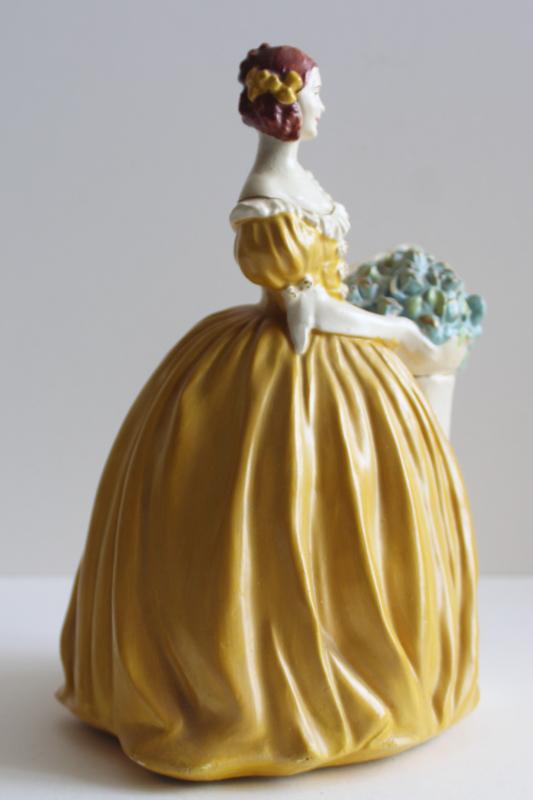The photograph captures a slightly blurry image of a miniature ceramic figurine of a woman in a voluminous, strapless yellow ball gown reminiscent of the 1800s. Her dress features white frills at the top and around its short sleeves, which terminate just below her forearms. The gown's billowy, ground-length design hides her legs entirely. The ceramic woman has chin-length, reddish-brown hair adorned with yellow bows, styled in a slightly curly manner. She stands in profile, revealing a serene smile and delicate facial features with red lips and a faint dot for an eye. Positioned beside or held by her is a white pedestal or bouquet holder filled with blue flowers, all part of the ceramic ensemble. The background includes a cream wall and a white table upon which the figurine is placed.